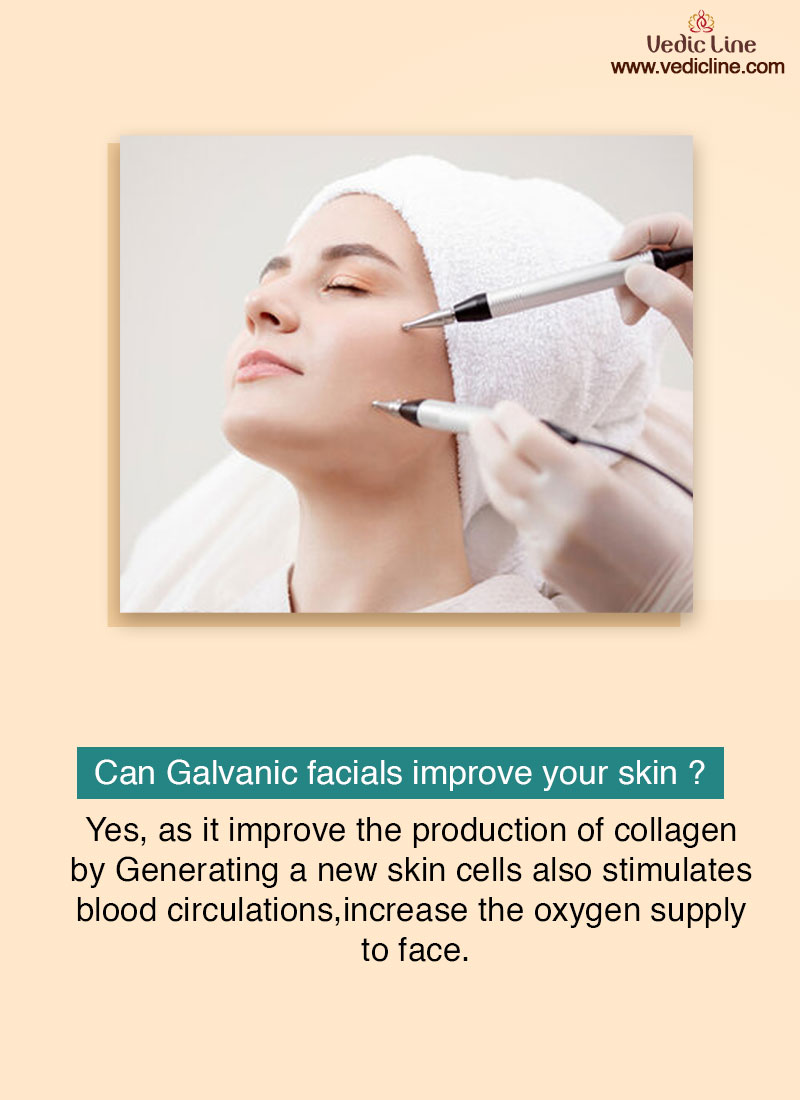The image features a woman undergoing a skin therapy treatment often referred to as a galvanic facial. She is wrapped in a towel covering her hair and part of her forehead, with her eyes closed and her head slightly tilted upward to the left. A medical professional, wearing white gloves, is using two pen-like devices with metallic tips, which are likely electrostimulation rods, and gently applying them to her cheeks. The background of the image is a light orange-pink hue. In the top right corner, there is a logo reading "Vedic Line" along with the URL "www.vedicline.com." Below the photograph, in white text on a turquoise rectangular background, it asks, "Can galvanic facials improve your skin?" This is followed by black text on the light orange-pink background stating, "Yes, as it improved the production of collagen by generating a new skin cells, also stimulates blood circulations, increase the oxygen supply to face." Although the text is written in somewhat broken English, it highlights the benefits of the procedure.